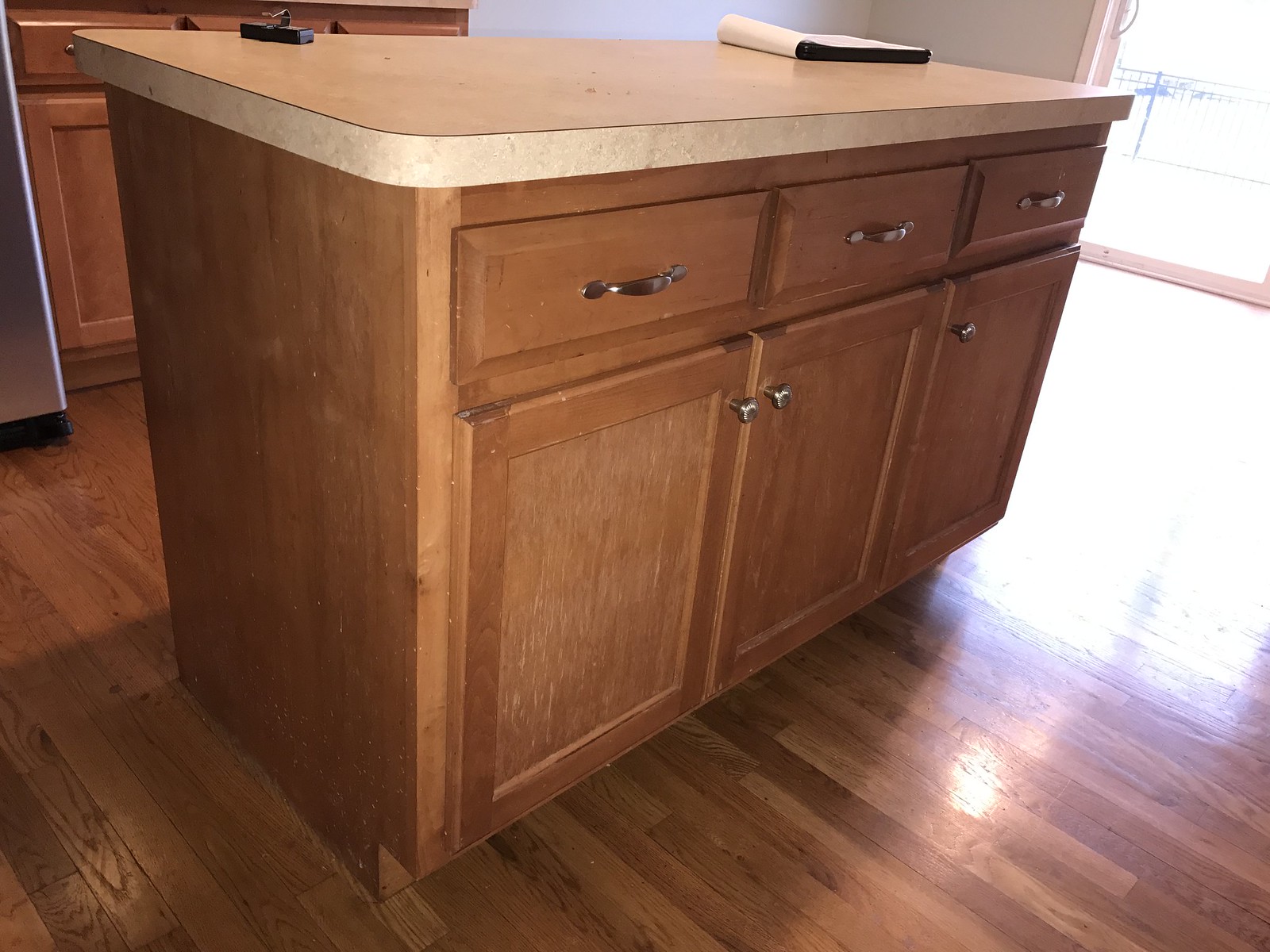The image features a centrally positioned kitchen island, surrounded by a sleek wooden floor that gleams under the sunlight streaming in from a nearby glass door. The island itself showcases a harmonious blend of functionality and aesthetics: its base is composed of rich brown wood housing three small drawers with brass or gold-colored handles, perfect for storing utensils. These are flanked by larger cabinets with matching knobs on either side, providing ample space for storing plates and bowls. The island's countertop is a creamy off-white surface, adorned with a notepad, and possibly a remote or a tray. Behind the island, a metallic refrigerator stands alongside additional drawers, enhancing the kitchen's modern yet warm ambiance. The natural light from the back door not only illuminates the room but also highlights the meticulous design elements of this inviting kitchen space.